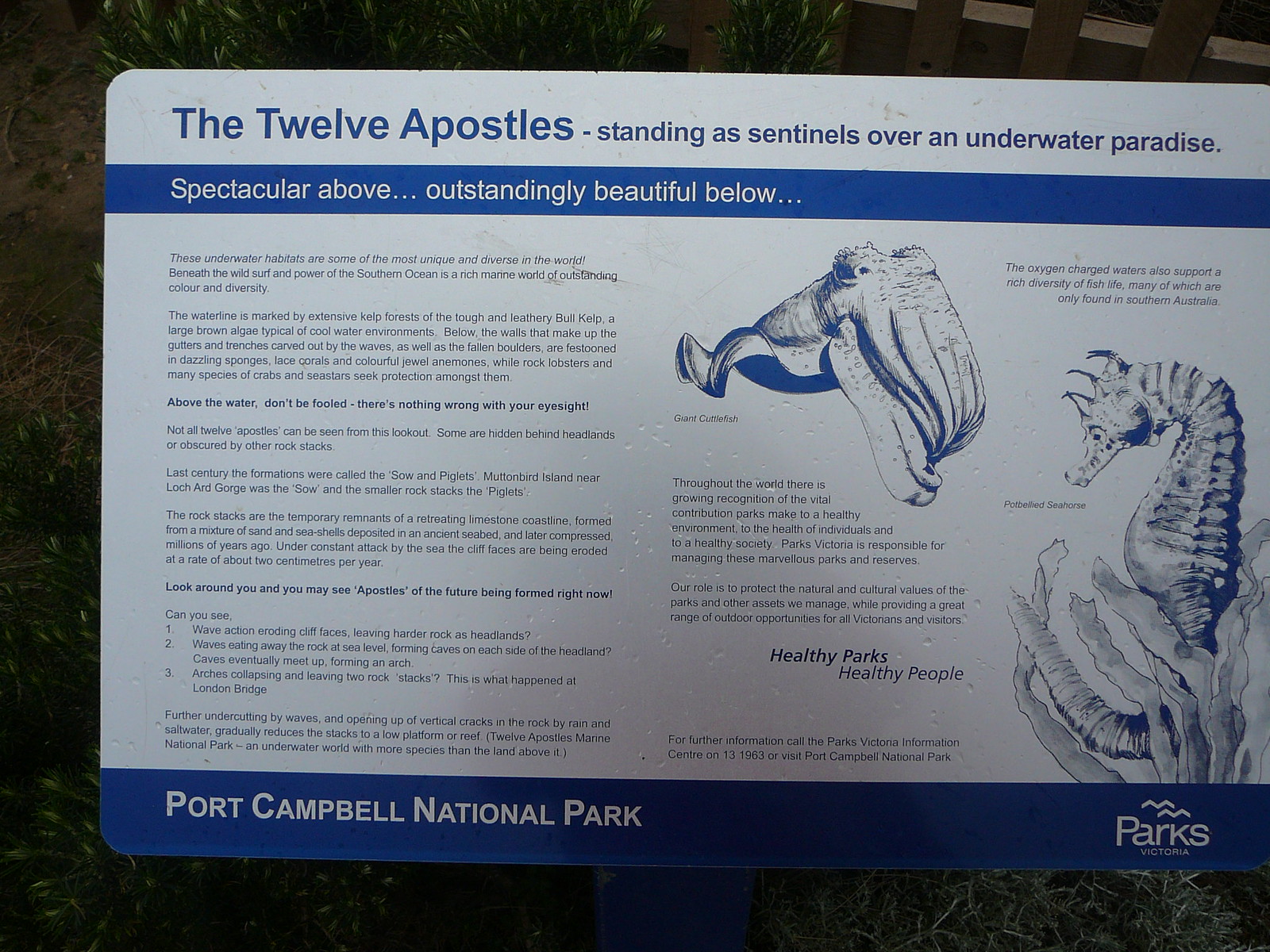This image captures a close-up of a detailed sign from Port Campbell National Park, labeled at the bottom with both the park's name and "Parks Victoria." At the top of the sign, bold text heralds "The 12 Apostles standing as sentinels over an underwater paradise." This striking phrase is followed by "spectacular above, outstanding, beautiful below," setting the tone for the description that follows. The sign's primary color theme is blue, with the majority of the text in varying shades of blue. To the right of the sign, illustrations of sea creatures such as a seahorse and a cuttlefish are prominently featured. The comprehensive text on the sign describes various animals that inhabit the marine environment, though it’s too extensive to read in full from the image. This detailed and informative sign seems more fitting for a museum or an educational exhibit rather than an animal enclosure or zoo.